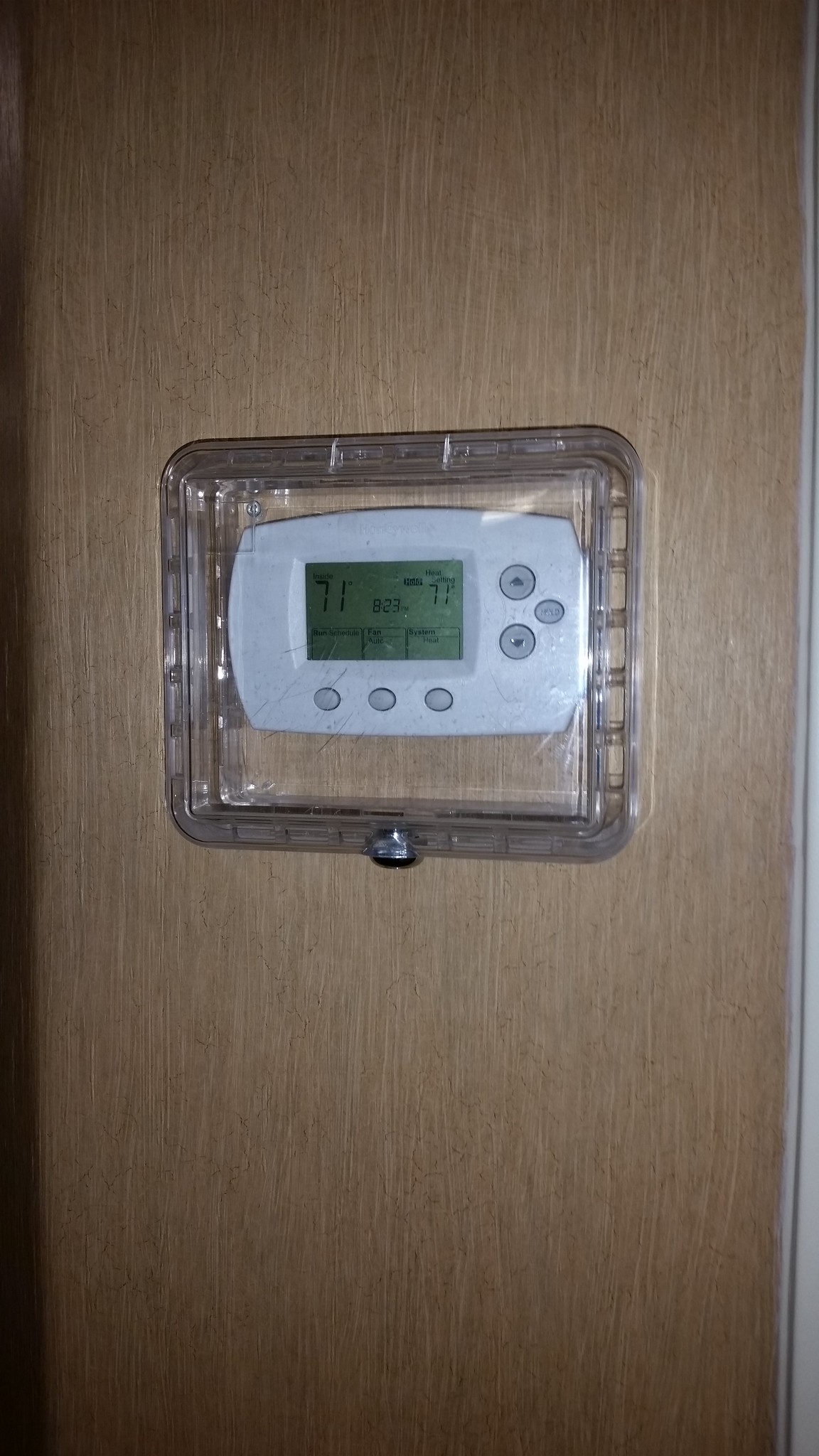The image features a wooden wall with a vertically oriented wood grain pattern, prominently showcasing a digital temperature gauge mounted at its center. The device is encased in a clear rectangular plastic cover that has a metal key opener at its bottom. 

The temperature gauge itself has a white border and includes three small gray buttons located along the bottom edge. On the left side, there are two larger buttons, and on the right side, there is a smaller button. The central feature of the gauge is its screen, which displays a primary reading of "71" and a smaller "71" on the right side of the screen. Although there is additional text visible on the screen, it is difficult to discern due to the wide angle of the shot.

Contextually, the right side of the image reveals a segment of another wall, beige in color, possibly indicating the presence of a doorframe nearby. The left side of the image is obscured by a dark shadow, adding contrast to the overall scene.